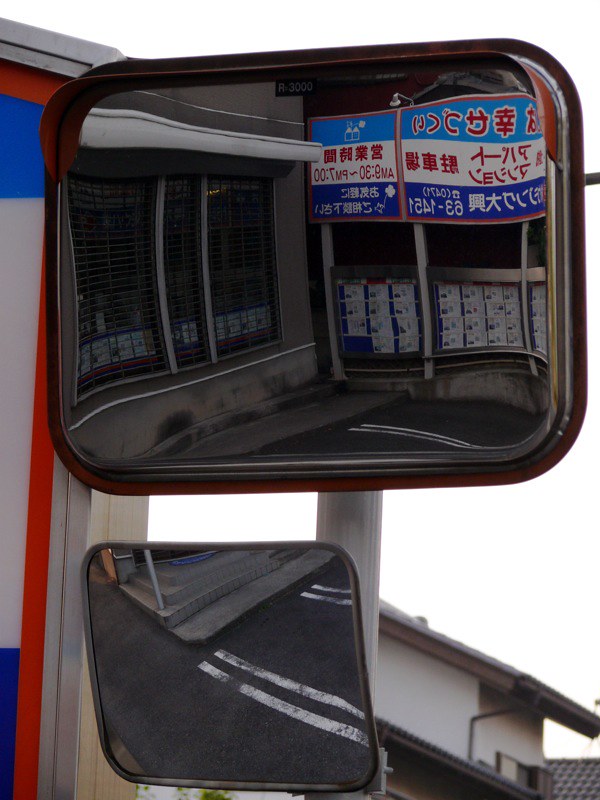The photograph captures two mirrors attached to a pole, reflecting their surroundings. Both mirrors feature Asian, likely Chinese, writing, though it is unreadable and appears reversed in the reflections. The mirrors seem to be mounted on the side of a vehicle, possibly a truck or van, colored in red, white, and blue—predominantly white. The setting is an outdoor urban area with an overcast sky. The backdrop includes a gray brick building and an asphalt pavement, possibly part of a parking lot marked with white lines. In the distance, there's a white building with a narrow, sloping roof, adorned with a window equipped with blinds and a white awning. The mirrors, particularly the smaller one, also reflect additional elements such as the street and sidewalk.